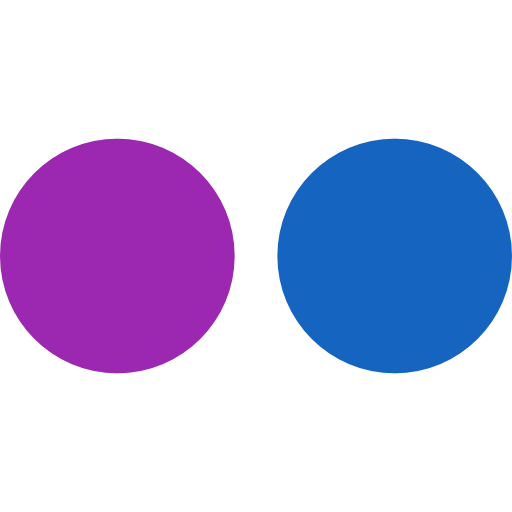On a plain white background, presumably a screenshot from a photo editing or paint application, two medium-sized circles are positioned side by side. They are spaced approximately an inch to an inch and a half apart. The circle on the left is a medium dark purple, while the circle on the right is a medium dark blue. Each circle is slightly larger than a half-dollar coin, creating a striking contrast against the stark white backdrop.